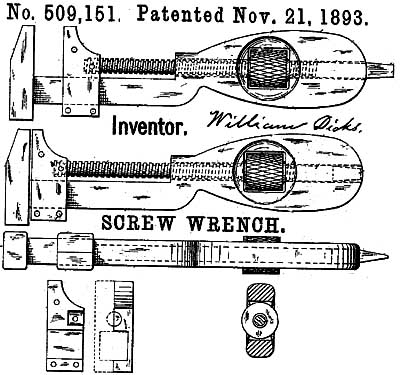This black and white illustration depicts a patent for a screw wrench, labeled "No. 509,151, patented November 21st, 1893." The inventor, William Dix, is credited between the top two illustrations. The image shows three views of the wrench: the first two views depict the wrench in an identical position, with the top image showing the wrench's opening expanded and the bottom image showing it closed. A screw runs through the middle of the wrench, protruding to the right in the top image and retracted in the bottom image. There is also an object within a hole in the screw designed to turn it. Beneath these, the words "screw wrench" are inscribed between the middle and lower images. The lower image presents the wrench lying on its side. Further, the bottom section of the illustration showcases the individual components of the wrench, including the pieces for its opening mechanism and an end-on view of the screw's threaded end. The precise black line drawings with no shading convey the technical design details clearly, emphasizing the functionality and construction of this heavy-duty clamping tool.